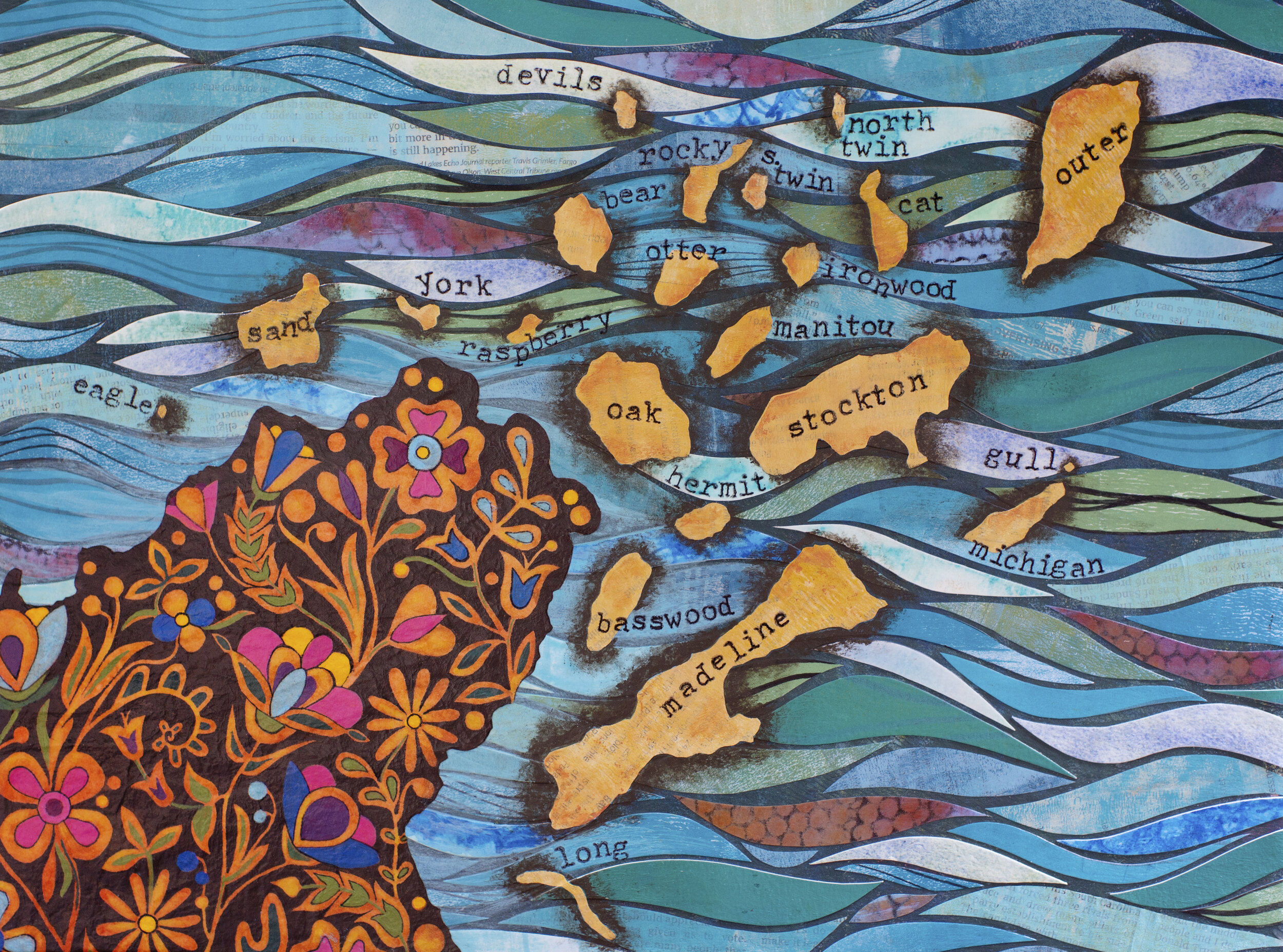This is a detailed artistic map drawing featuring a series of landmasses, possibly islands, each labeled with names such as Stockton, Oak, Madeline, Outer, York, Sand, Eagle, Devils, North Twin, Rockies Twin, Cat, Otter, Ironwood, Manitou, Raspberry, Hermit, Basswood, Gullo, Michigan, Long, and Bear. These names are written in black text amidst a vibrant, wavy background composed of interwoven hues of blue, teal, red, white, and green, accented by black outlines. While the exact nature of these landmasses is unclear, they rest atop a backdrop that resembles vast, undulating waves. Adding a touch of intricate detail, the bottom left corner of the image features a striking floral design with a black background adorned with colorful flowers in shades of orange, pink, blue, green, purple, and yellow, creating a rich, eye-catching contrast against the wave-patterned expanse.